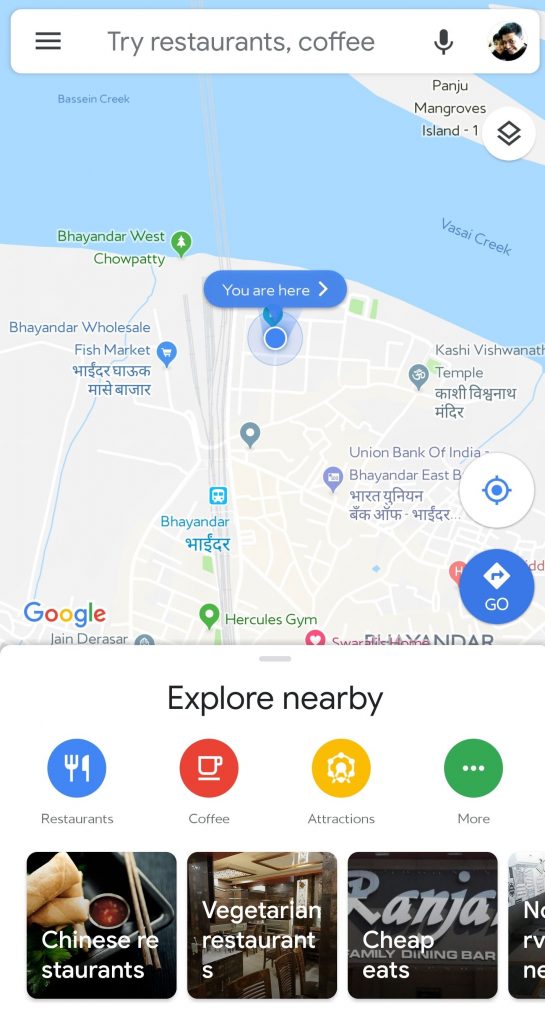A Google Maps screen is displayed, featuring a user's profile picture in the top right corner. The image in the profile picture appears to show the user with a child, who could possibly be their son, daughter, or nephew. At the top of the screen, there is a search bar along with a microphone icon for voice searches.

A map marker has been placed on the map, which is focused on a location in India, as suggested by visible Hindi text and local names such as "Vaishwanath Temple" and institutions like the "Union Bank of India." At the bottom of the screen, there is an "Explore Nearby" section offering various categories such as Chinese restaurants, vegetarian restaurants, and cheap eats. Additional options are available, enabling the user to explore restaurants, coffee spots, attractions, or more by clicking an aptly labeled "more" button.

Visible map elements include a layers button, which likely offers various map views such as topographical information. Other map features include options to readjust the compass or get navigation directions. The Google logo can be seen on the bottom left, confirming that this is indeed a Google Maps interface.